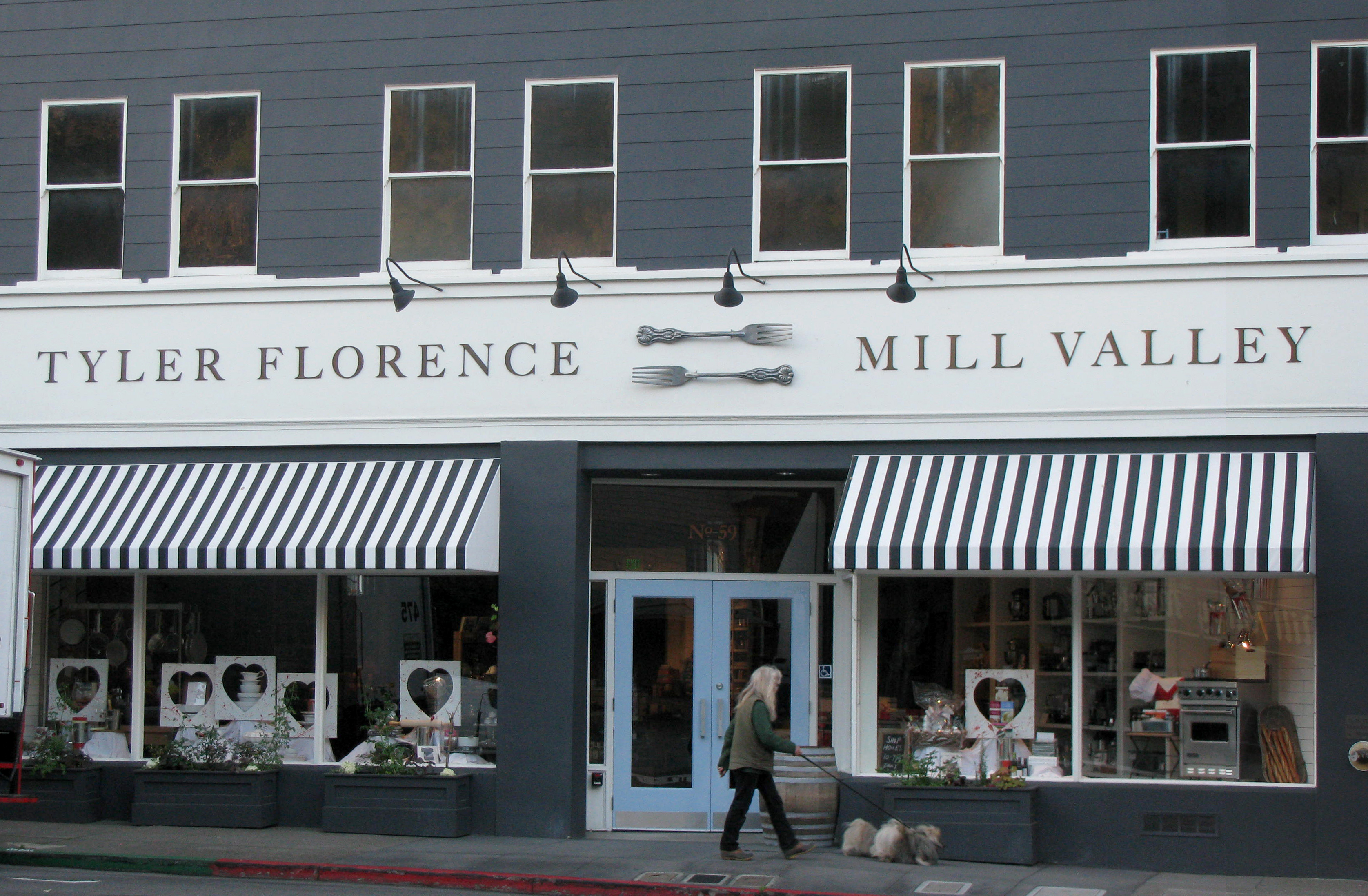This image features a stylish storefront with blue siding, prominently displaying a sign that reads "Tyler Florence" accompanied by graphic design elements of two forks pointing in opposite directions. To the right of the sign, "Mill Valley" is written in gray font on a white background. Above this sign, there are four sets of paired square-paned windows, making for a total of eight windows. Adding to the ambiance, four flood lamps are positioned to illuminate the sign.

Below the sign, the building showcases elegant white and blue pinstriped awnings, which are situated diagonally and transition to a vertical orientation at the lower section. These awnings cover the windows and doorways, with one awning on each side of the establishment—one under "Tyler Florence" and the other beneath "Mill Valley."

The lower portion of the storefront consists of three windows to the left, two windows to the right, and two central glass doors topped with a vertical glass transom. The windows offer a glimpse into the store, which contains displays of heart-shaped frames and an array of kitchen appliances and decorative items, hinting at a culinary-themed shop.

In front of the store, a woman with blonde hair is walking her dog on a leash, both facing towards the establishment. The scene is picturesque, capturing the essence of a quaint, well-decorated shopping destination.